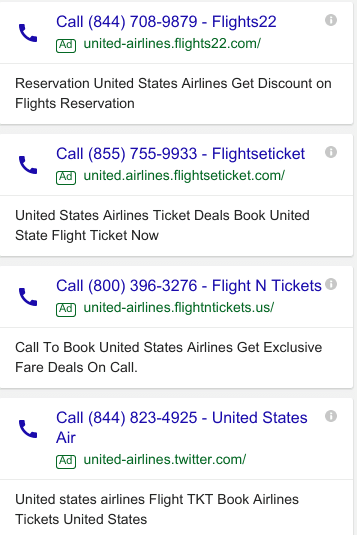The image displays a Google search results page with the top four entries marked as ads. Although the specific search query isn't visible, it's evident that the results pertain to flights. Each of these top four ads is identified with a small green square labeled "Ad" and all are from or associated with United Airlines. 

The ads point to two distinct websites selling United Airlines tickets, differentiated primarily by their contact phone numbers. Here's a detailed breakdown of the ads:

1. **Top Ad:** Ends with "flights 22". The description emphasizes reservations with United States Airlines and mentions discounts on flights.
2. **Second Ad:** Ends with "flights ticket". Similar focus on reservations and flight discounts.
3. **Third Ad:** Ends with "flights and tickets". The description follows the same theme as the previous ads.
4. **Fourth Ad:** Ends with "United States Air". 

At the bottom of these ads, there's another ad that states: "United States Airlines flight TKT, book airlines tickets United States." This ad appears unusual and possibly foreign due to its unconventional phrasing.

Overall, all ads promote the idea of reserving discounted flights with United Airlines, though their presentation varies slightly.